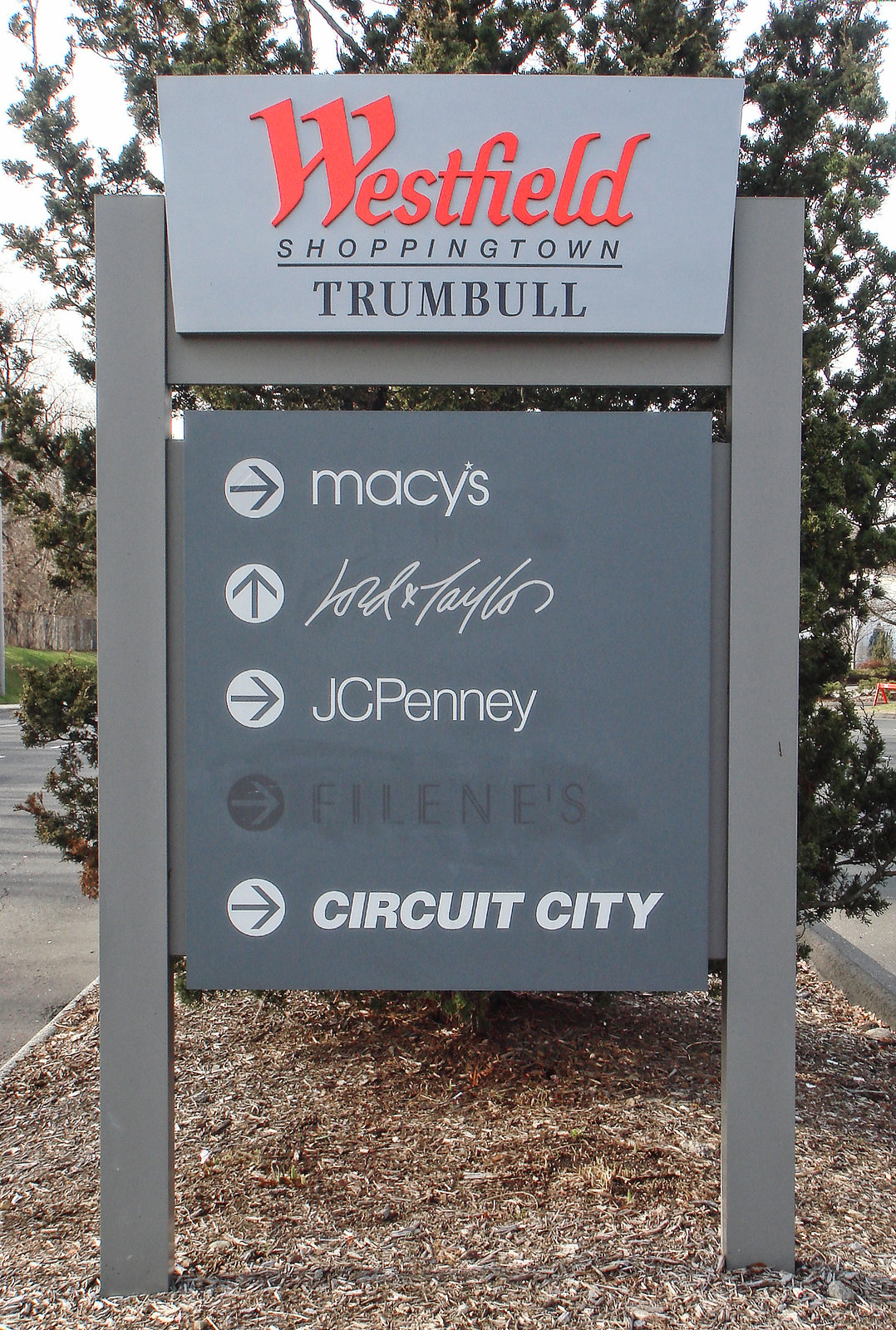At the entrance of the Westfield Shopping Town in Trumbull, a large, dark slate-colored sign offers directions to various stores. Positioned in a bed of mulch surrounded by shrubbery, the sign serves as a divider for incoming and outgoing traffic. It directs shoppers to Macy's, JC Penney, and Circuit City to the right, while Lord and Taylor is straight ahead. Notably, a darker gray section lists "A. Leans," which is difficult to read compared to the other store names in white. This detailed signage ensures visitors can easily find their favorite stores within the mall.